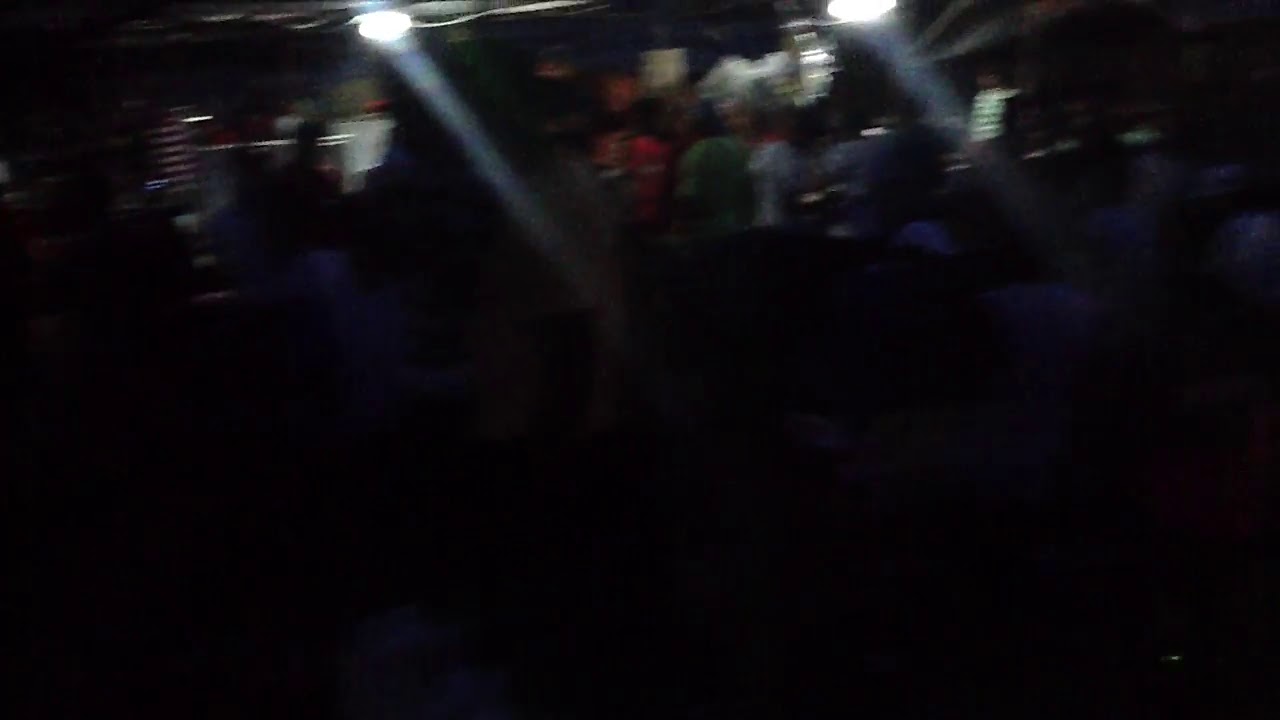This image is a very blurry and grainy photograph taken in a dark setting, making it difficult to discern specific details. The scene appears to depict a large gathering of people with their backs to the camera, possibly at an event such as a concert or sporting occasion. Toward the top of the image, two lights shine downwards, partly illuminating the scene. The colors visible in the photo include black, white, gray, green, red, orange, silver, light blue, and brown. Due to the poor quality and darkness, the surroundings and exact nature of the event remain indistinguishable, and no text or clear objects can be seen apart from the general crowd and lights. Some horizontal lines off to the left suggest the presence of stairs, but this is not definitive. Overall, it is an indoor scene with the main elements positioned towards the top center of the image.